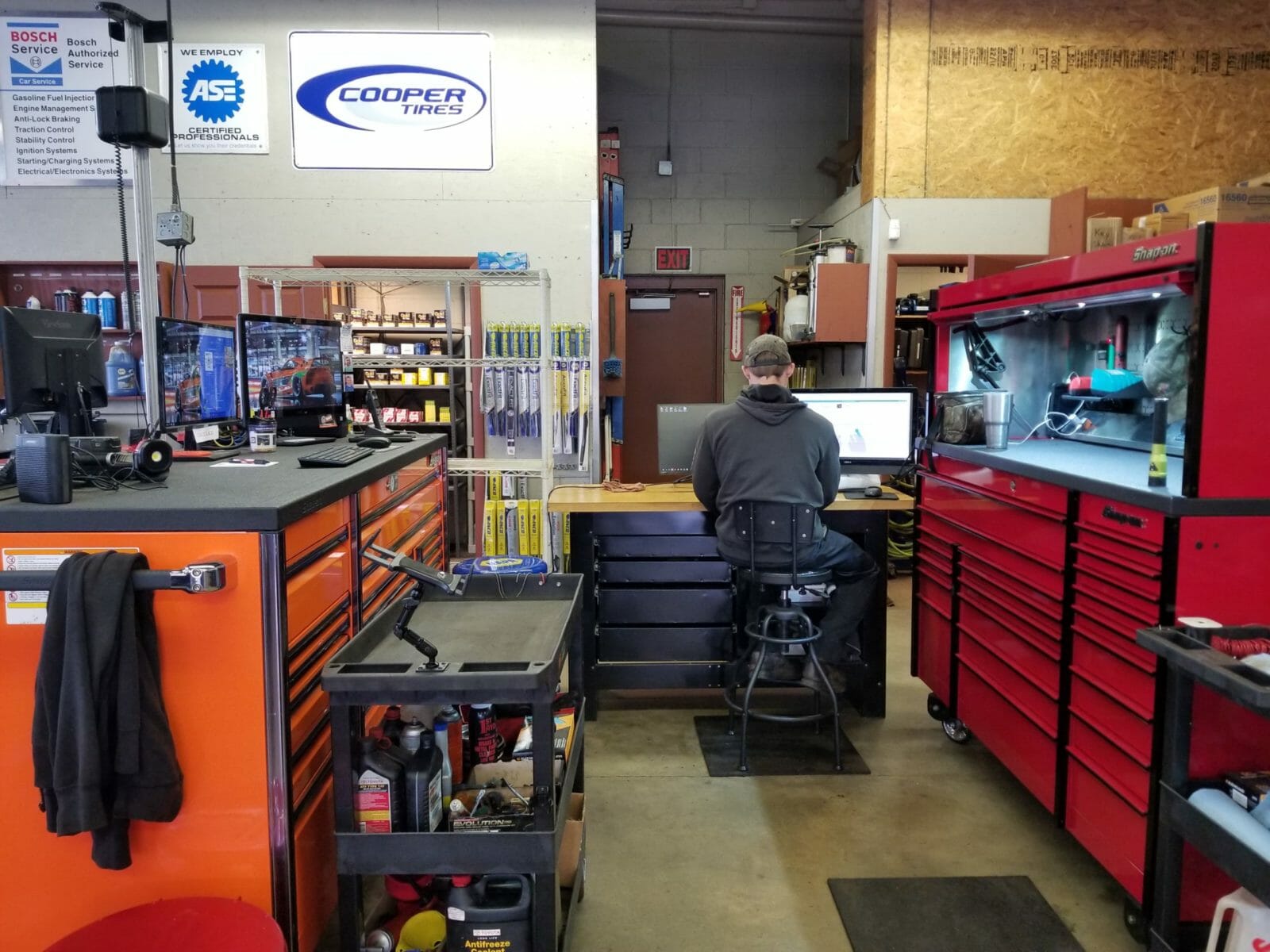In the image, a person is seated in a mechanic shop, focused on their work. They are wearing a gray hoodie, a greenish hat, dark pants, and black boots, and are sitting on a brown chair. The individual is using a computer setup consisting of two monitors, one white and one black. The backdrop is a gray cement cinder block wall, featuring a red exit sign positioned above a brown door. Adjacent to the door is a red arrow pointing downward towards a red fire extinguisher. To the right side of the person is a red tool case, containing a lighting fixture and a grayish mug. 

The top right section of the image shows a gray plywood wall, while the left side features a whiter plywood wall with several signs. One sign reads "Cooper Tires" with a blue circle above it, and blue font. Another sign says "ASC" in white font within a blue circle with ridges on its perimeter. To the left of that is a sign for "Bosch Service" with blue font on a white background. Additionally, there is an orange tool station with a black countertop and more computer monitors near the individual. A black coat or sweater is draped over a black pole, and a black, three-shelved wheeled rack is also visible in the garage.